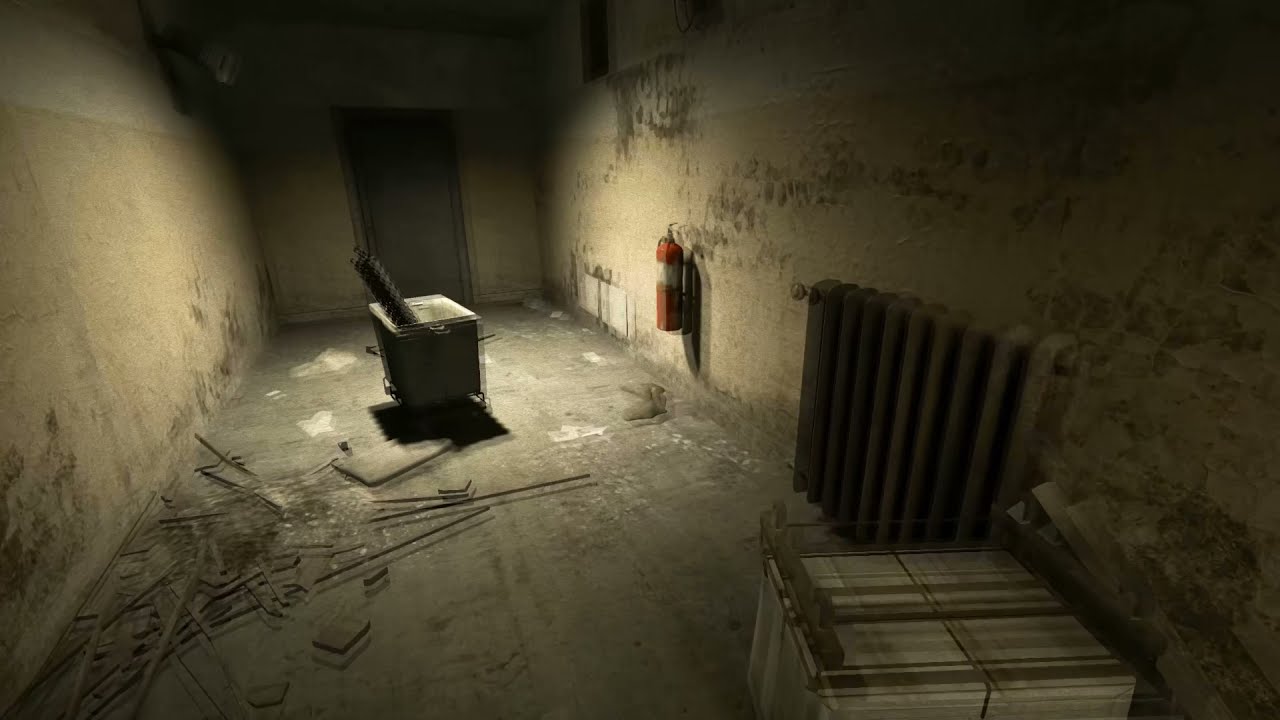This exceedingly out-of-focus and poorly lit image appears to draw inspiration from a horror video game, depicting a decrepit, rectangular room in notable disarray. The space is defined by its severely deteriorated state: beige and yellowing walls marred by peeling paint, with a white brick border evident at the top. Debris, potentially including wood molding and rocks, litters the gray floor, augmenting the room's chaotic atmosphere. 

The far end of the room is characterized by a shorter wall with a large closed gray door, evoking a sense of confinement. Central to the scene is a large, wheeled bin filled with dark, indeterminate contents—perhaps reminiscent of a trash bin or deep freezer without a lid. A red fire extinguisher, hanging a few feet off the ground on the right wall, is notably illuminated despite the dim lighting. In the foreground, an old-style radiator and a box are discernible among the scattered debris.

Overall, the blurred image, coupled with the dilapidated condition of the room and its ominous contents, crafts a vivid narrative of abandonment and decay.